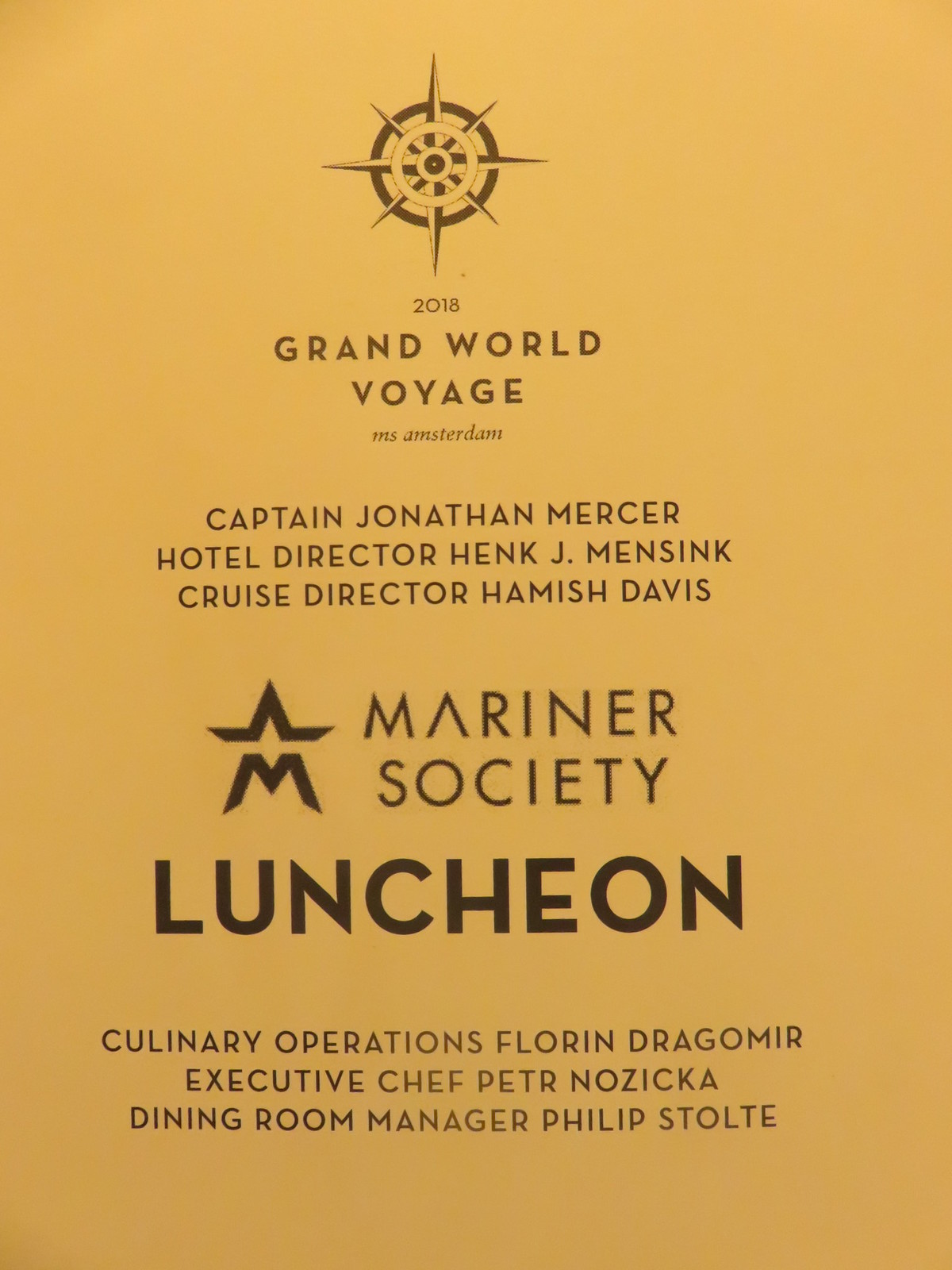The image showcases a vividly yellow poster featuring a detailed announcement for the "2018 Grand World Voyage" aboard the MS Amsterdam. At the top, an eight-pointed compass and the year "2018" set the stage. The main text reads "Grand World Voyage" in large black capital letters followed by "MS Amsterdam" in lowercase. Highlighted prominently are key personnel: Captain Jonathan Mercer, Hotel Director Henk J. Mensink, and Cruise Director Hamish Davis. Beneath, the "Mariner Society" is accompanied by a star-shaped logo to its left. Bold and capitalized, the word "Luncheon" stands out, indicating a special event. Further details list Culinary Operations managed by Florine Dragomir, Executive Chef Petar Nozica, and Dining Room Manager Philip Stoltz. The overall design of the poster is striking, using bold black text against a yellow background to convey the information clearly.